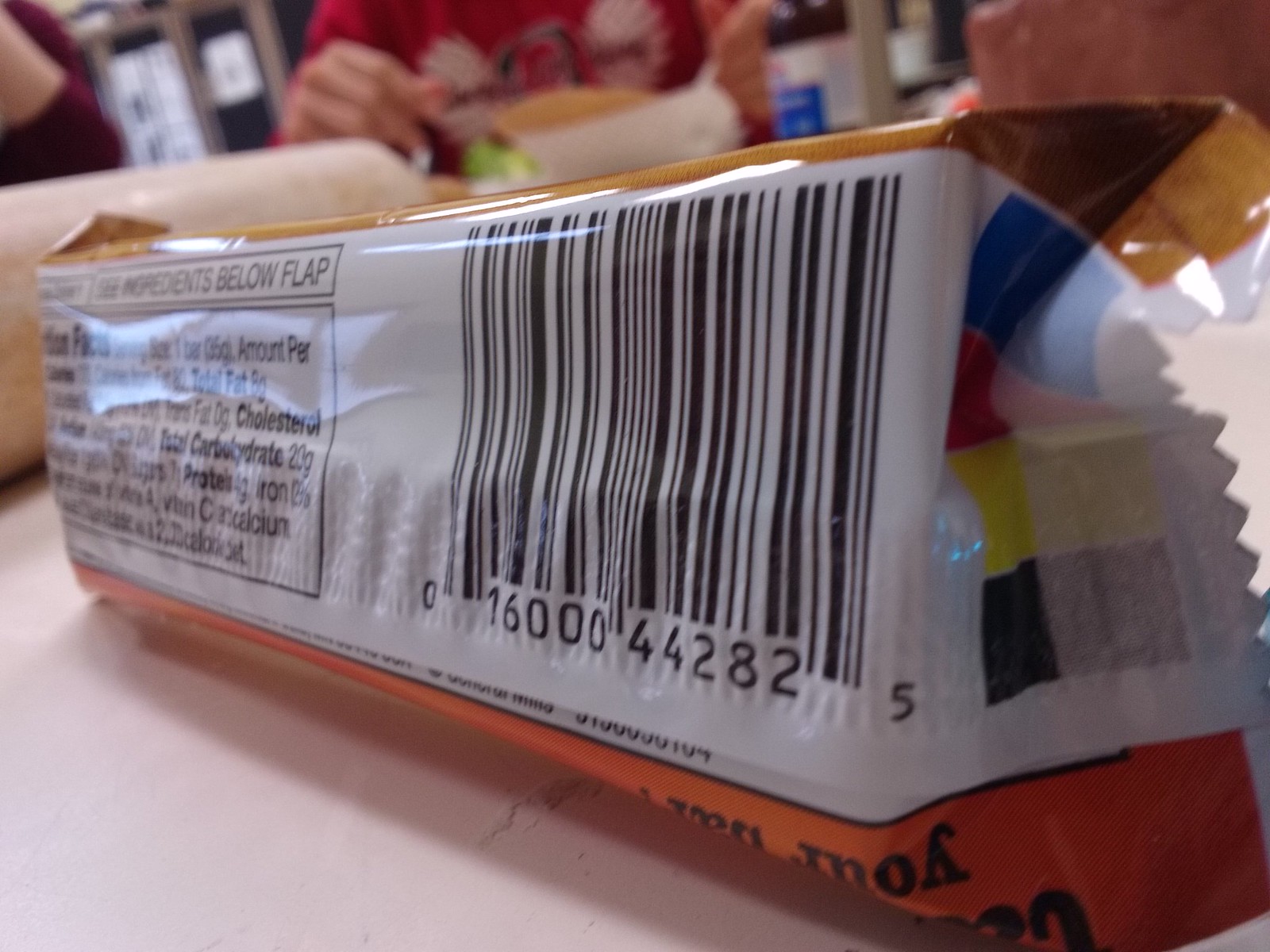This color photograph features the back of an individually packaged rectangular snack bar, with a prominent focus on its plastic wrapper. The bar is positioned on a white table at an angle, making the barcode, 016000442825, the most visible element on the right side, while the nutritional facts are on the left but are blurred and hard to read due to glare. The wrapper features a light brown color on the top and transitions to orange at the bottom, with the word "YORE" partially visible upside-down near the bottom. A color-coding bar with blue, red, yellow, and black rectangles is present at the end of the wrapper. In the blurred background, there are people seated at the same table with other food items. The composition is free of any animals, plants, buildings, or vehicles.